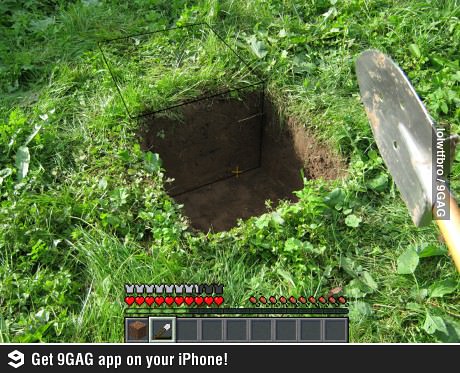The image is a digital photograph of a real-life scene in a grassy field, with green grass and weeds surrounding a precise, square-shaped hole dug into the ground, mimicking a Minecraft block of dirt. The square hole is central to the composition and highlights a cube-like space in the earth. An augmented reality overlay imitates the Minecraft user interface, featuring a cubic border above the hole to indicate a player's viewpoint and the customary HUD (Heads-Up Display) at the bottom. The HUD shows partially full health hearts, a shield icon, and full food bar indicators resembling meat icons with white bones. Moreover, there are nine inventory slots, one of which contains a real-life shovel that has a silver blade and a brown handle. Additional elements include a small black textbox saying "LOL WTF BRO / 9GAG" and a black strip at the bottom reading "Get 9GAG app on your iPhone?" in white font.